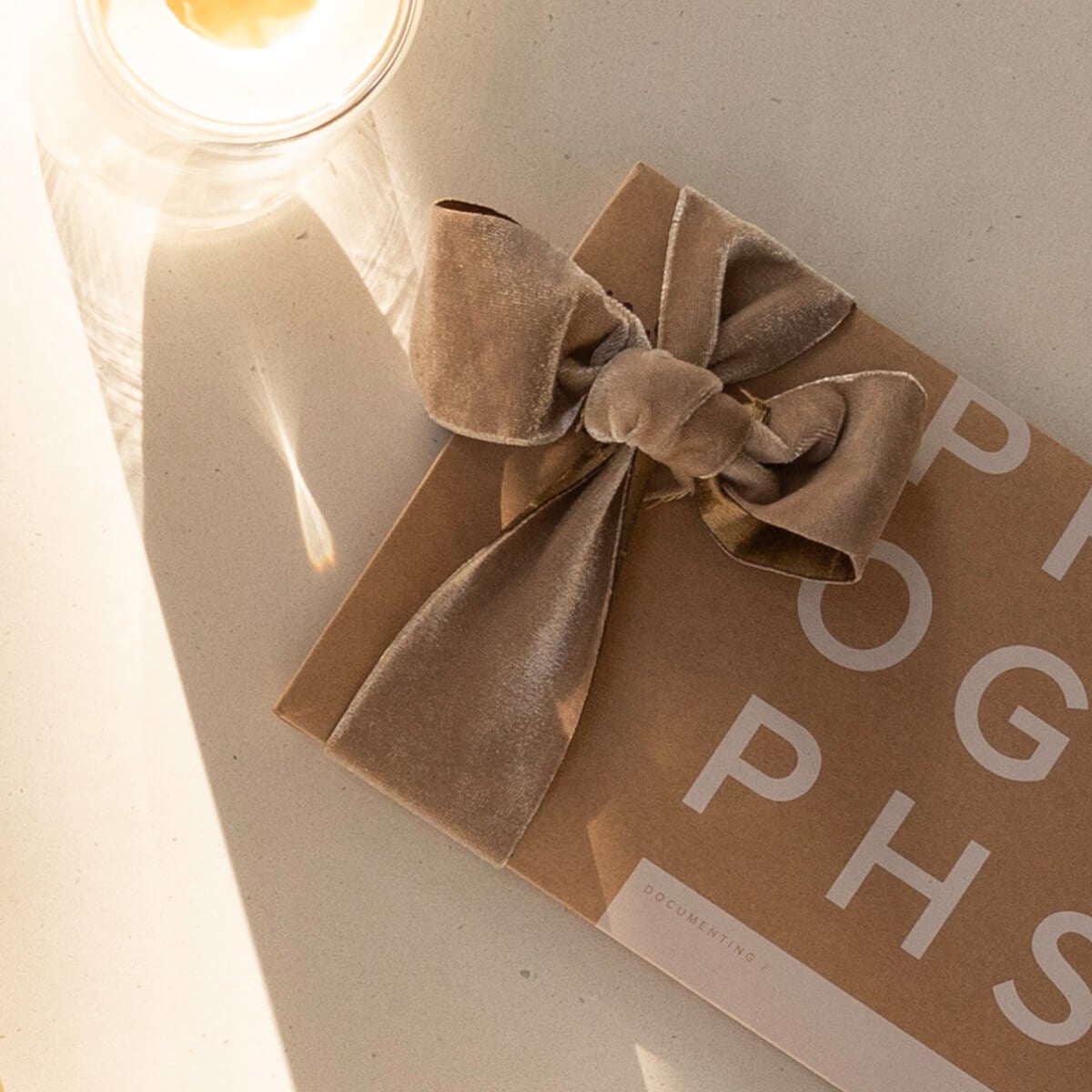The image displays a partially visible brown envelope positioned on a light gray surface. Decorated with large white letters spelling "P I O G P H S," the envelope is wrapped with a taupe-colored velvet bow or ribbon on one side. Emphasizing the elegant presentation, the thick felt bow adds a luxurious texture to the package. The background features a soft, whitish, textured surface. In the upper left corner, an illuminated circular bulb shines brightly, casting reflections and a prism-like glow onto the background, enhancing the serene and delicate ambiance of the scene.